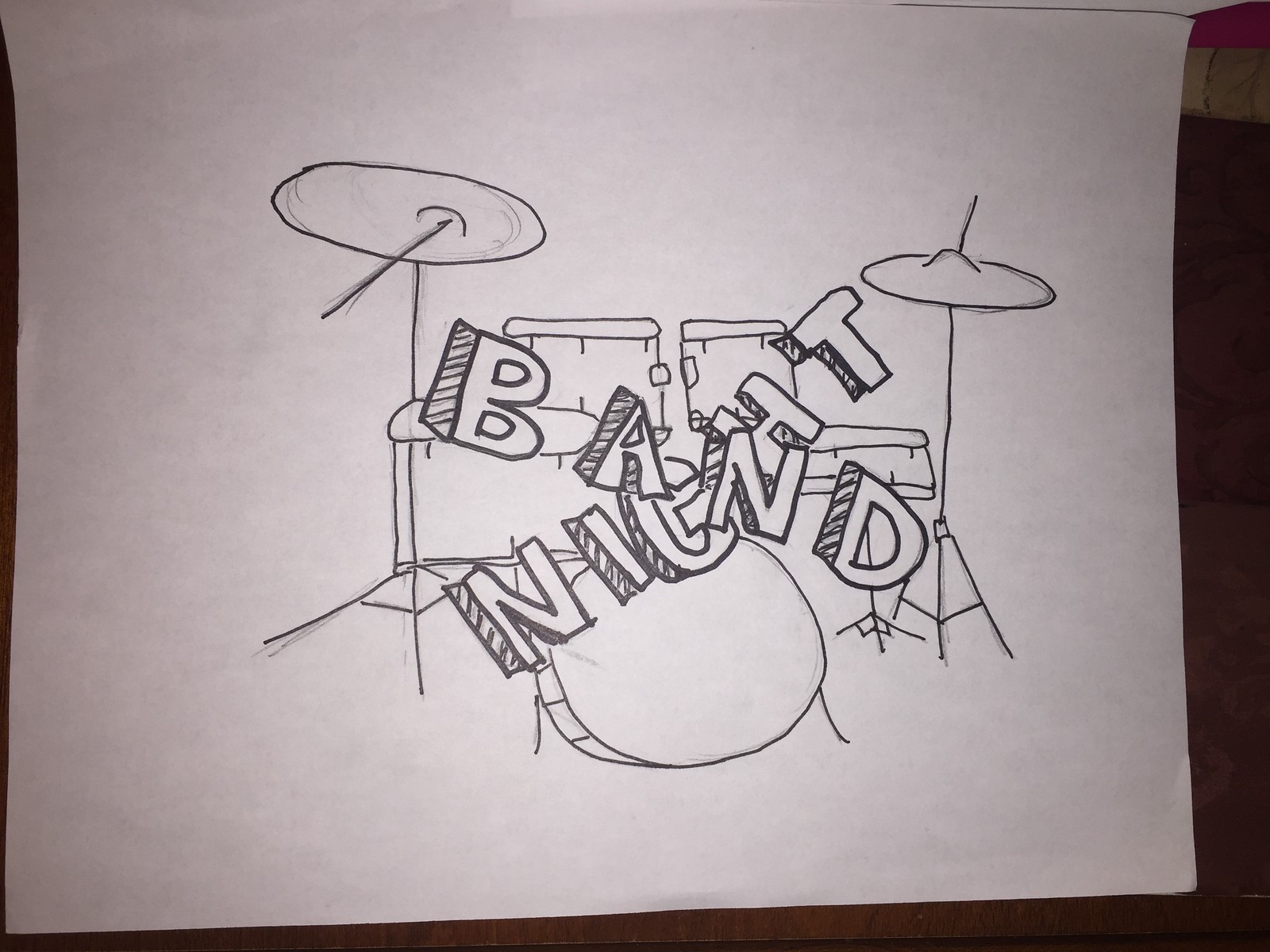This photograph captures an 8.5 by 11-inch piece of white paper laid out horizontally, featuring a crudely sketched drum set drawn solely in pencil without any added colors. At the center, two primary drums are positioned towards the back, flanked by a pair of cymbals on either side, depicted as circles supported by straight lines with additional lines for the base. In front, a larger bass drum stands prominently with its legs splayed, contributing to the overall rudimentary representation of a typical drum kit.

Overlaid on the drum set are the bold, shaded block capital letters forming the words "BAND NIGHT," arranged in a crossed fashion—'Band' aligned diagonally from top left to bottom right and 'Night' from bottom left to top right. The 3D-like lettering adds a striking emphasis to the otherwise simple drawing. The entire composition, likely created by a younger individual or perhaps intended as a casual note or advertisement for a band event, is presented against an indeterminate background, emphasizing the spontaneous and personal nature of the sketch.